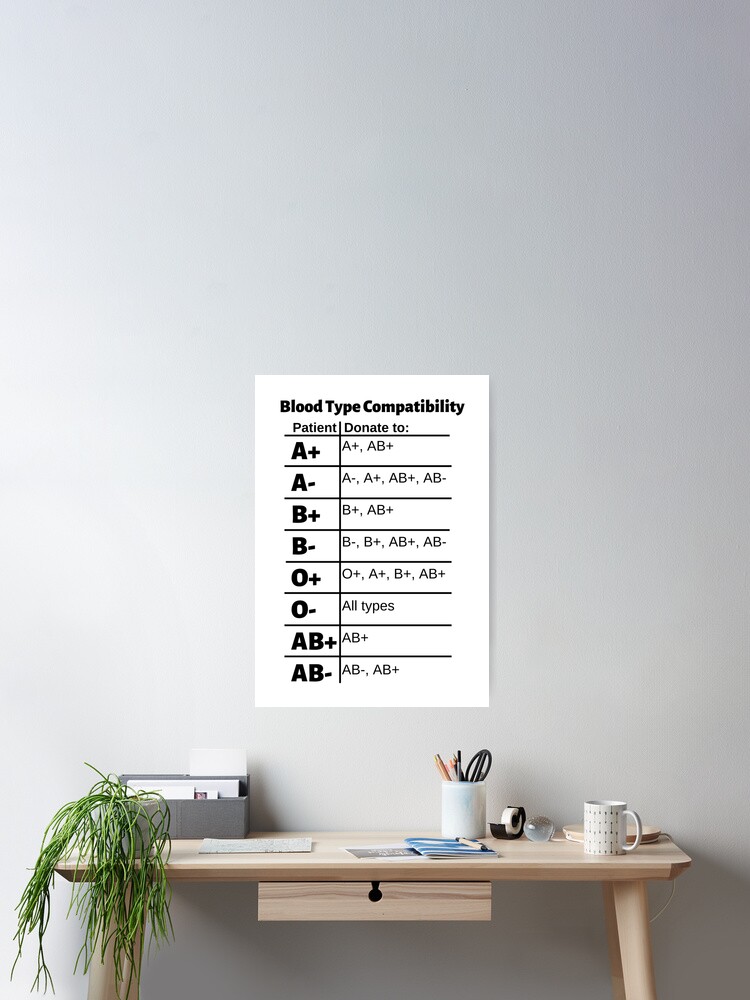In a brightly lit room, presumably within a doctor's office or hospital, a small white poster prominently displaying "Blood Type Compatibility" is affixed to an off-gray wall. Detailed information is printed in black, listing various blood types and their compatibility for donations: 

- **A positive (A+)**: compatible with A+ and AB+
- **A negative (A-)**: compatible with A-, A+, AB-, and AB+
- **B positive (B+)**: compatible with B+ and AB+
- **B negative (B-)**: compatible with B-, B+, AB-, and AB+
- **O positive (O+)**: compatible with O+, A+, B+, and AB+
- **O negative (O-)**: compatible with all types
- **AB positive (AB+)**: compatible only with AB+
- **AB negative (AB-)**: compatible with AB- and AB+

Below this informative poster, there is a wooden desk featuring several organized items: on the left side, a small pot containing a plant; on the right side, a flexible white desk lamp. Also on the desk are a white mug filled with scissors and pencils, a tape dispenser, and a mail container. This setup includes the functional and minimalistic tools frequently found in healthcare environments.